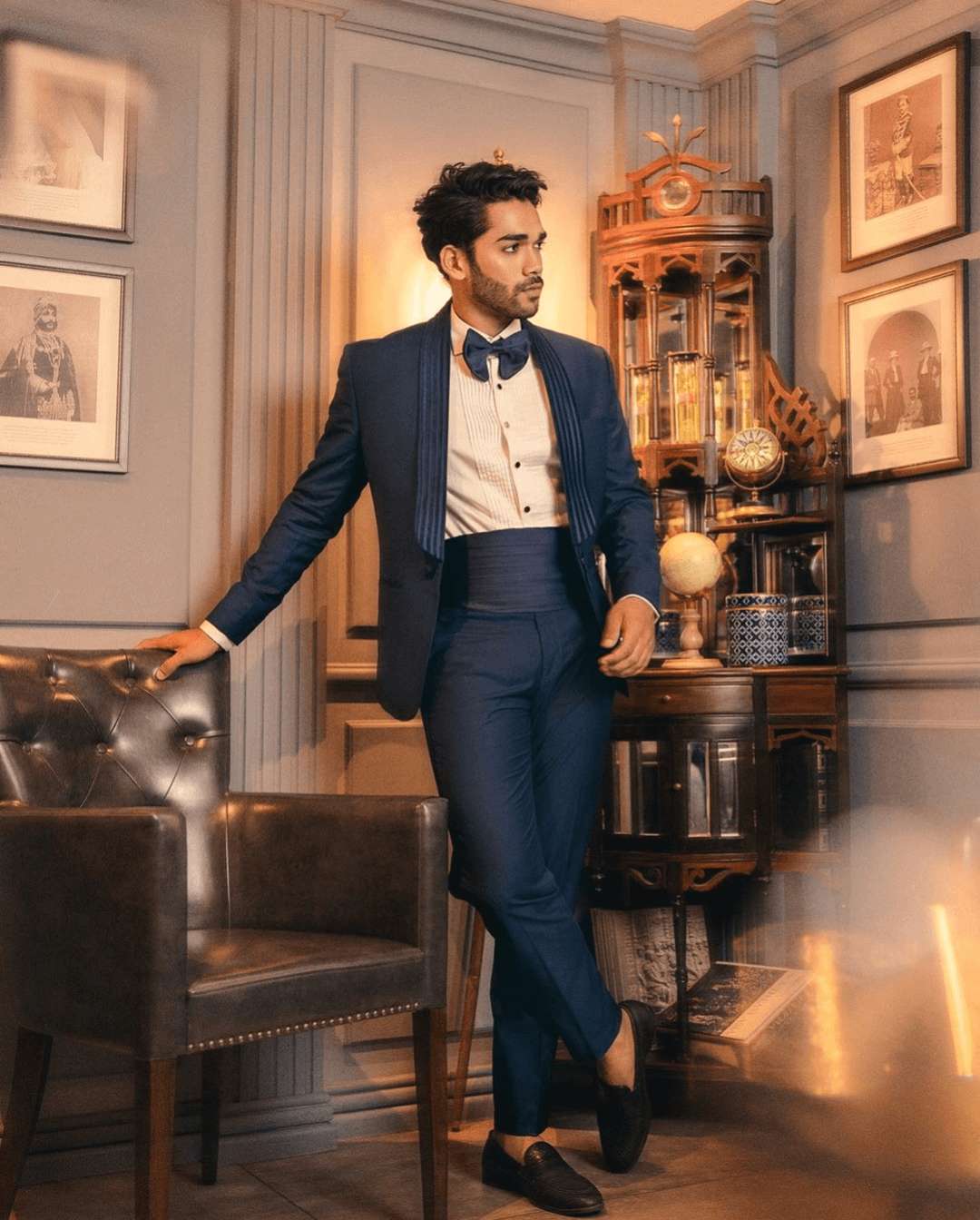The image depicts a dark-skinned man with short brown hair and a slight bearded mustache, wearing a blue tuxedo ensemble that includes a blue jacket, a white shirt with a blue bow tie, and blue pants. His outfit is completed with black or dark brown shoes, notably worn without socks, and a distinctive blue sash around his waist. The man stands in a room resembling a living room, leaning with his right arm on a silver or black leather chair, with his left hand positioned in front of him. 

He gazes to the right of the frame while his body faces forward, with his right leg crossed over his left. The background features a light gray-blue wall adorned with four pictures. The two pictures on the right side of the man hang beside a wooden armoire or cabinet; the top picture is slightly out of focus, and the bottom picture portrays a person from a bygone era. To the left and behind the man, the other two pictures can be seen, adding to the vintage ambiance of the space. Near the armoire, a wooden semi-circle desk is cluttered with various ornaments and silver and gold objects. The overall composition suggests a past era with a mix of old-time photographs and furniture, evoking a sense of nostalgia.